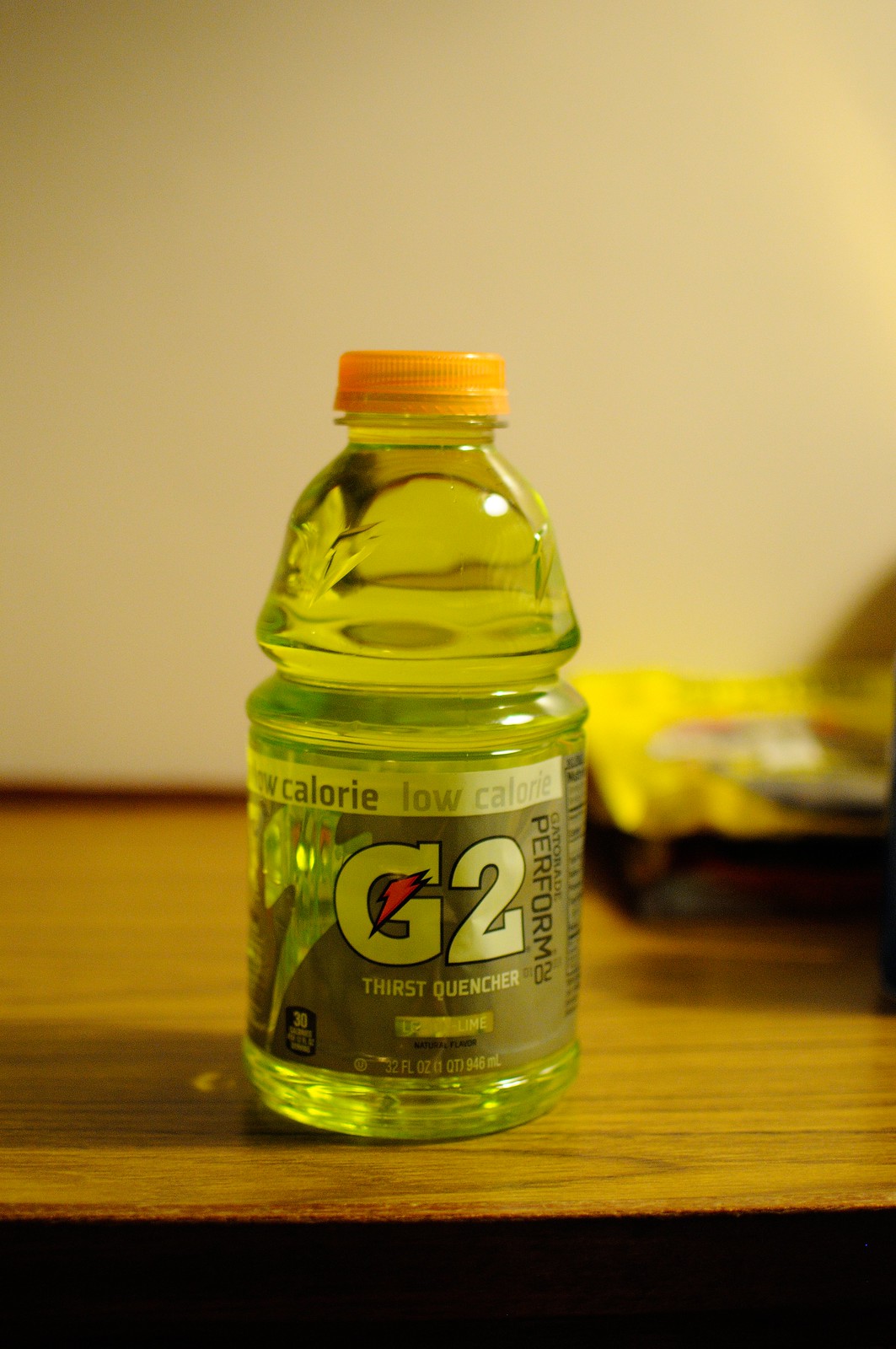A Gatorade bottle filled with a translucent yellow liquid sits prominently on a wooden surface, likely a table. The table's top features a brown hue with a darker wood grain running through it, and it appears slightly stained. The bottle is topped with an orange cap. The bottom half of the bottle showcases a label with "G2" emblazoned in white letters with a black outline, featuring the Gatorade lightning bolt incorporated into the "G". Above "G2," there is black text that reads "Gatorade performs," while below, "thirst quencher" is written in white. Additional details on the label include "32 fluid ounces" and a white strip at the top stating "low calorie." The background is blurred, revealing only indistinct objects to the right and a white wall behind them. The bottom edge of the image displays the black edge of the table.